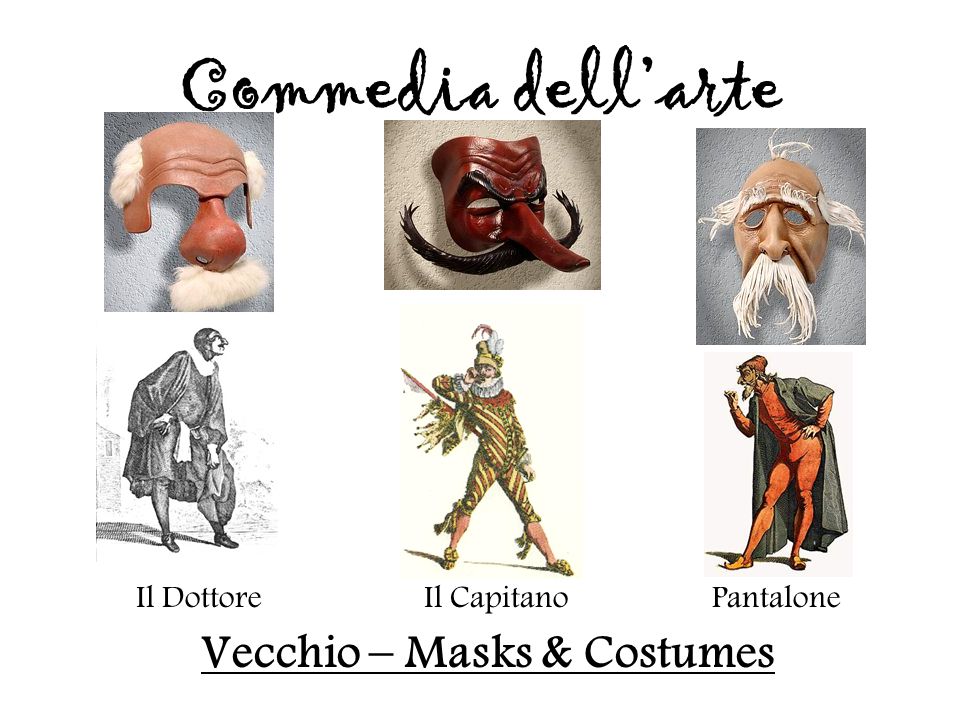The poster details three distinct types of "Vecchio" masks and the characters traditionally associated with them in "Commedia dell'Arte." The title at the top reads "Commedia dell'Arte," followed by a subtitle "Vecchio Masks and Costumes." The layout consists of three columns and two rows, making a grid of six images against a solid white background. 

The top row features photographs of masks: 
1. The left mask depicts an elderly man with a wrinkled forehead, white hair on the sides, a large nose, and a white mustache. Below it, a black-and-white sketch of a character wearing the mask is labeled "Il Dottore."
2. The middle mask is red-faced with a long nose, curly mustache, and pointy eyebrows, conveying an intense expression. Beneath it is a colored sketch of a character labeled "Il Capitano," depicted wielding a sword and dressed in a gold-striped and red outfit.
3. The mask on the right has a droopy face with a long, droopy mustache, stringy white hair above the ears and white fur on top. Below, a colored sketch labeled "Pantalone" shows the character in an orange unitard with a cape.

The bottom row consists of these corresponding character sketches, each associated with the mask above it, reiterating the classical costumes and personas of these "Commedia dell'Arte" figures.